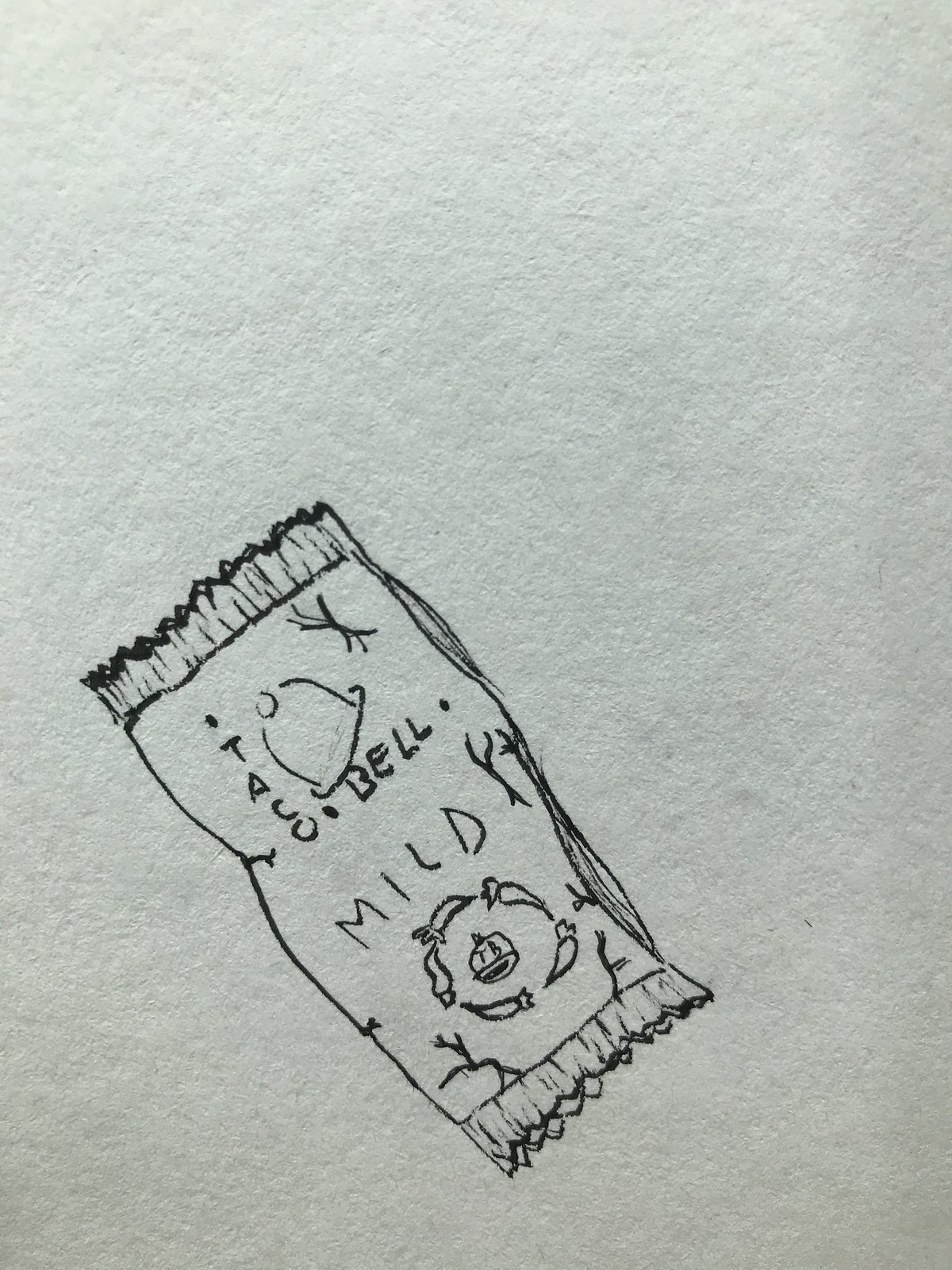A meticulously detailed black pen drawing captures an angled view of a Taco Bell mild hot sauce packet. The packet is positioned towards the bottom-left of the paper, but the paper's edges remain unseen due to the camera's close-up focus on the sauce packet. The illustration faithfully replicates the packet's details, with the words "Taco Bell" rendered in precise pen strokes, alongside a finely outlined bell emblem. The word "mild" stands prominently in pen above the packet's signature diagram, which features peppers encircling the word "mild." The artist has skillfully shaded several creases to give the packet a lifelike texture, all accomplished through detailed pen work.